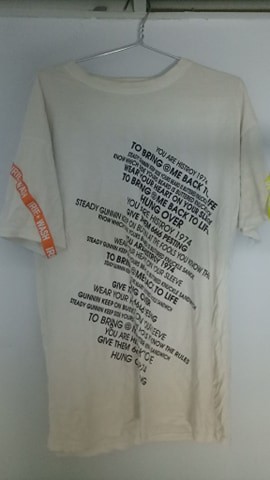The image depicts a vintage, yellowish-white t-shirt hanging on a wire hanger with a traditional triangle shape, set against a faded white wall. The t-shirt has noticeable wrinkles and creases, particularly towards the bottom. Central to its design is a pattern of black text extending from the chest down to the navel area, printed slightly crooked—angled about 10 degrees to the right. This text appears in bold and lighter variations, featuring phrases such as "You are history" and "1974," although some words are obscured by the fabric's folds. The right sleeve is adorned with an orange sticker or tag that reads "pre-wash" in white text. The photo, seemingly taken from a first-person perspective on a phone, captures the t-shirt hanging from a wire clothes hook, adding to the image's casual, authentic feel.